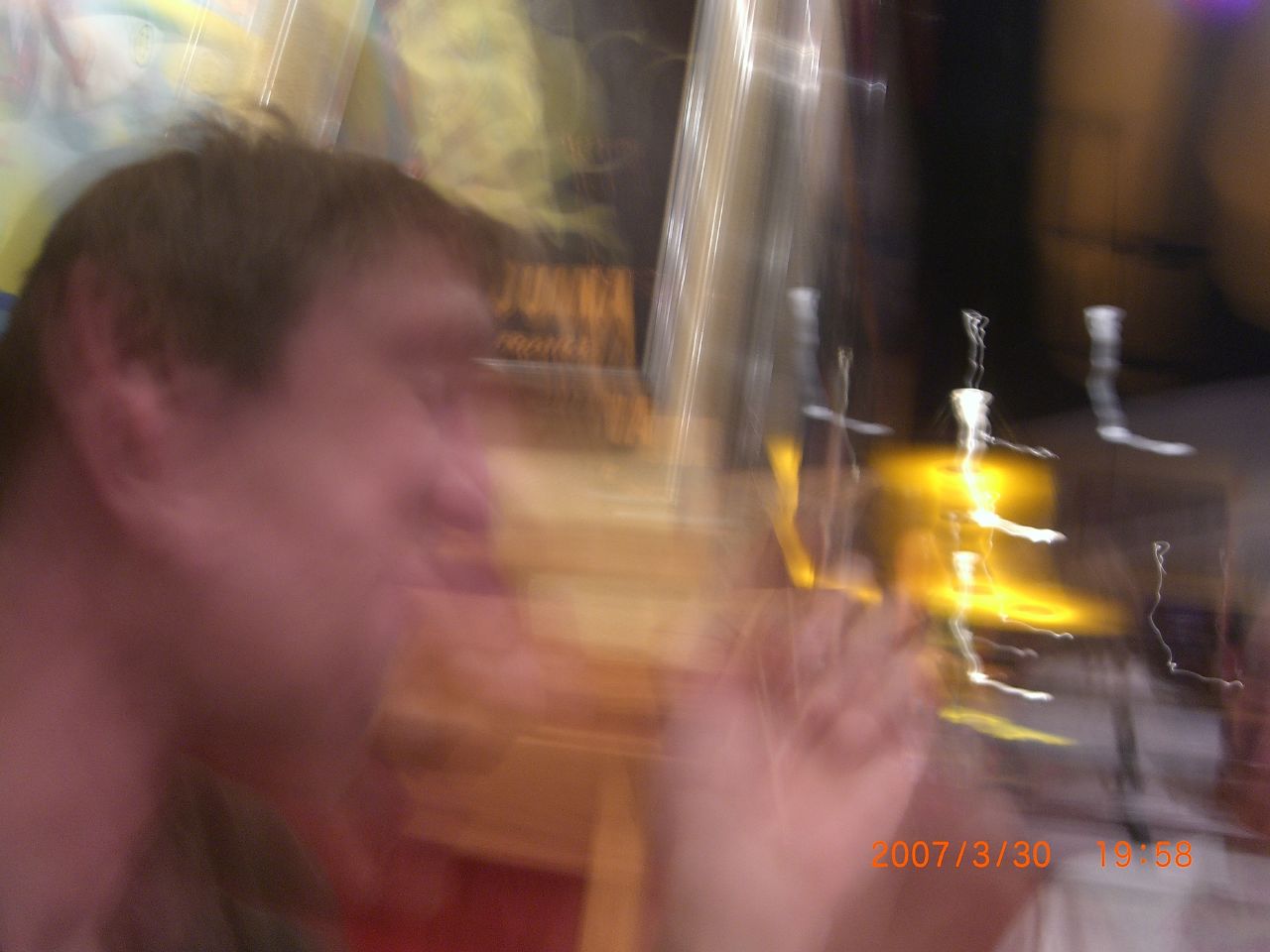This photograph, dated March 30, 2007, at 19:58, captures a blurry image of a man. Despite the lack of clarity, certain features are discernible. The man has short brown hair, a white neck, and no facial hair, with his ear, nose, eye, and mouth faintly visible. One of his hands is raised, adding to the scene’s dynamism. He appears to be standing outside a shiny, possibly metallic, yellow object, although it is unclear whether this object is a car, a building, or something else. The intentionality behind the blurriness remains uncertain.